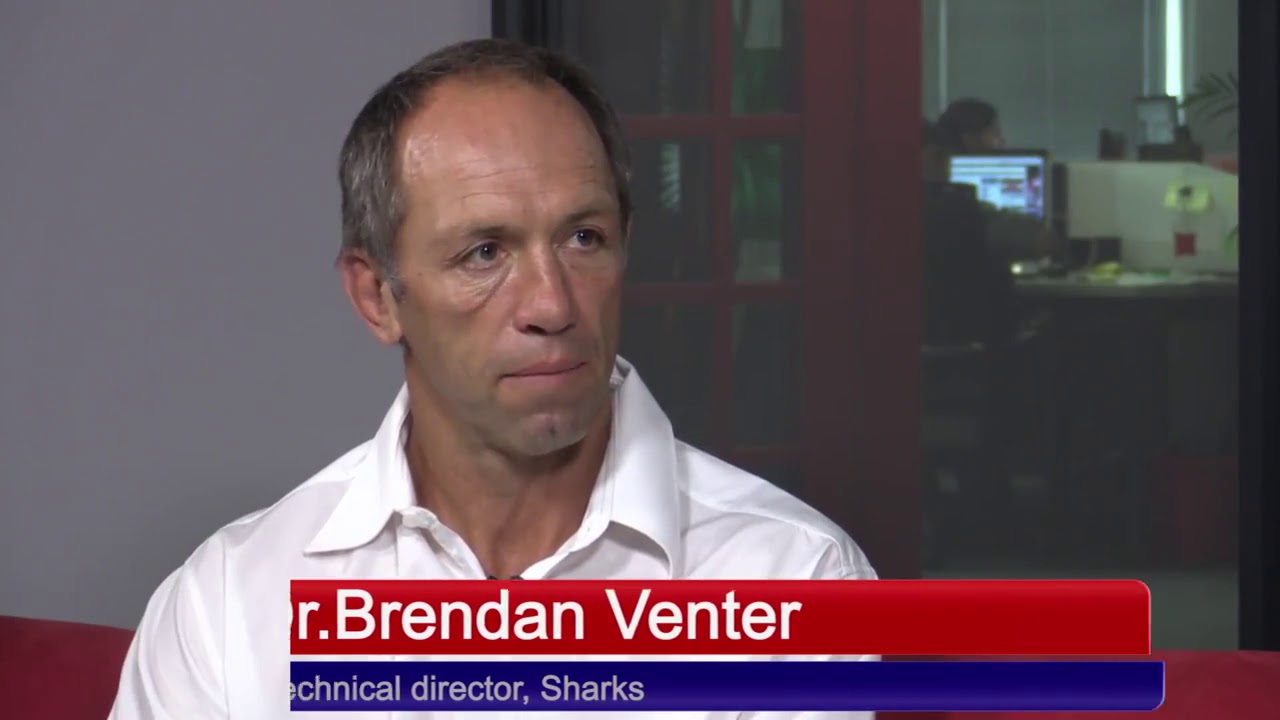The image is a still frame from a news report featuring an older, serious-looking gentleman with gray hair and slight bags under his eyes, wearing a white long-sleeve collared dress shirt. He appears to be in an office setting, with a red-framed wooden door with glass windows behind him, through which an office area with people working on computers is visible. The background includes a whitish-gray wall to the left and sunlight peeking in on the top right corner, along with a small flower next to the computers. The image is partly covered by text identifiers: "R. Brendan Venter" written in white font on a red stripe, with the "D" cut off, and below that, "technical director, sharks" in white font on a blue stripe, with the "T" also cut off. The man is looking slightly to his right.